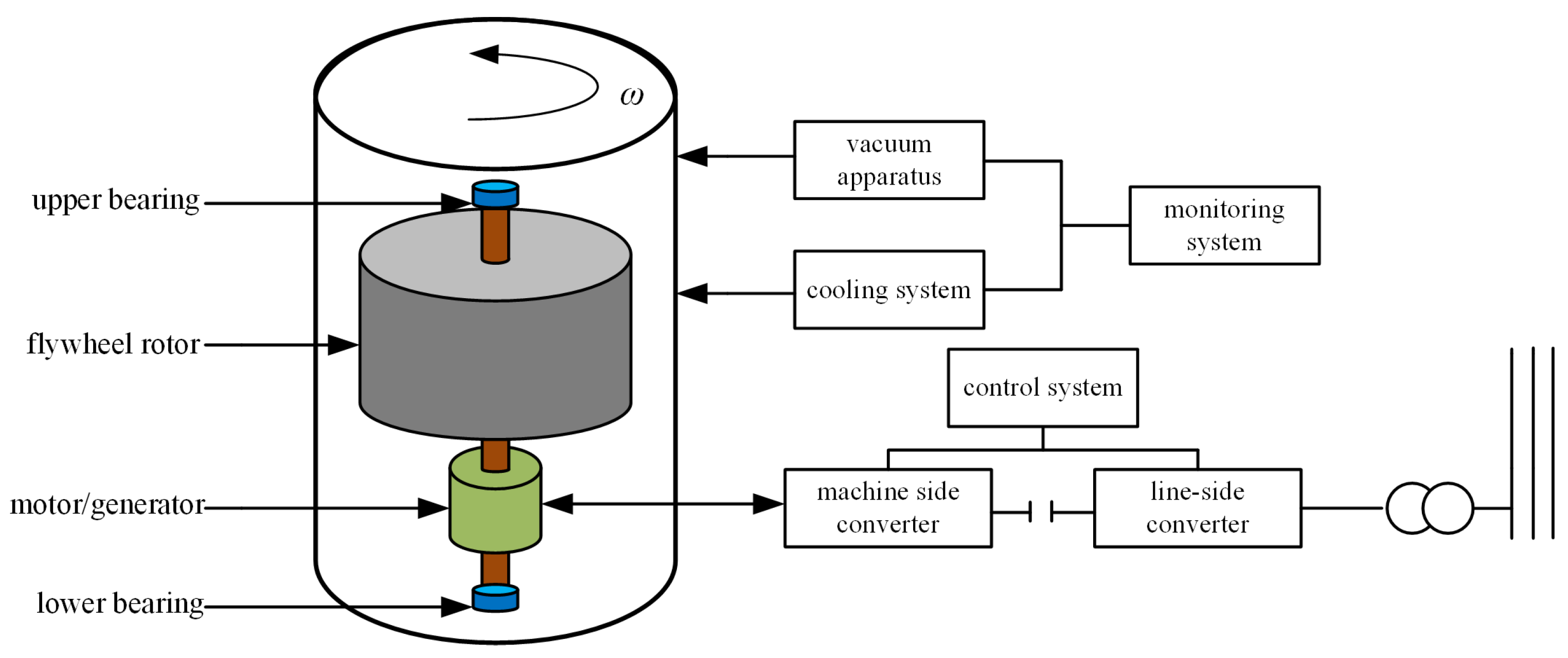This illustration is a detailed diagram of a mechanical device, likely found in instructional manuals for mechanical engineers. Central to the drawing is a large, transparent cylinder, depicted in outline with black, containing several key components. At the center of the cylinder is a prominent gray wheel, identified as the flywheel rotor. Below it is a smaller green wheel marked as the motor generator, with blue caps at both the top and bottom labeled as the upper and lower bearings, respectively. A brown shaft runs through the middle, connecting these parts. Surrounding the device, labeled pointers indicate the functions of different systems: a vacuum apparatus, a cooling system, a monitoring system, a control system, a machine side converter, and a line side converter. The diagram serves to detail the intricate components and their interactions within the motor encased in the cylinder.